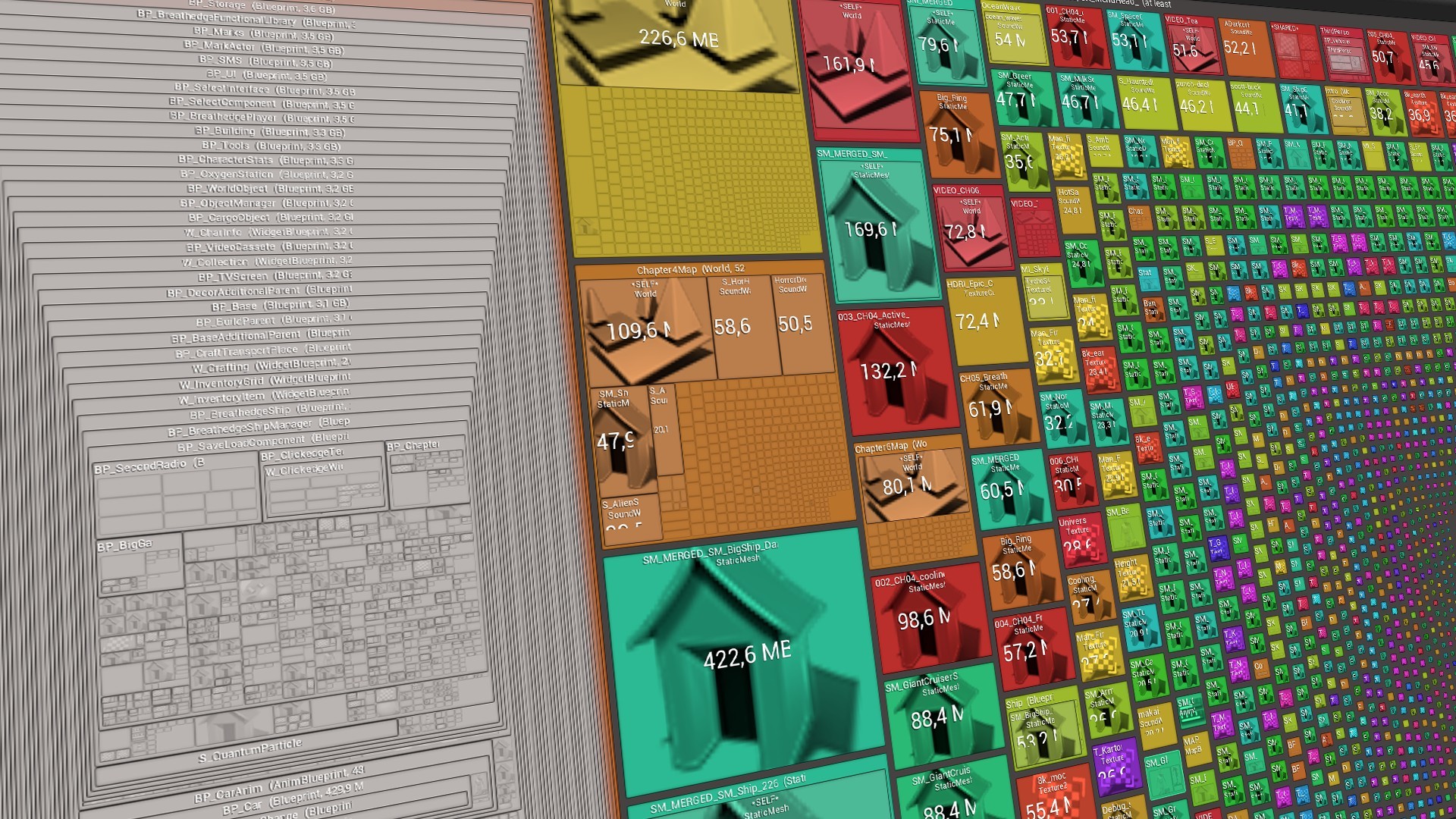The image appears to be a vibrant and intricate digital mosaic resembling a user interface from a video game or shopping site. The mosaic features a grid of multicolored squares—yellow, orange, blue, red, green, and purple—each depicting various small housing structures like shacks, outhouses, and sheds. These squares decrease in size towards the bottom right corner, becoming tiny pixels. The larger squares are interspersed with smaller ones, adding to the abstract yet fascinating aesthetic. On the left side of the mosaic, there's a grayish area that resembles an entryway or a pixelated structure, suggesting it might be part of a virtual world the player can navigate. The repeated patterns and numbers on the squares give the entire piece a diagrammatic feel, making it a complex and captivating piece of digital art.